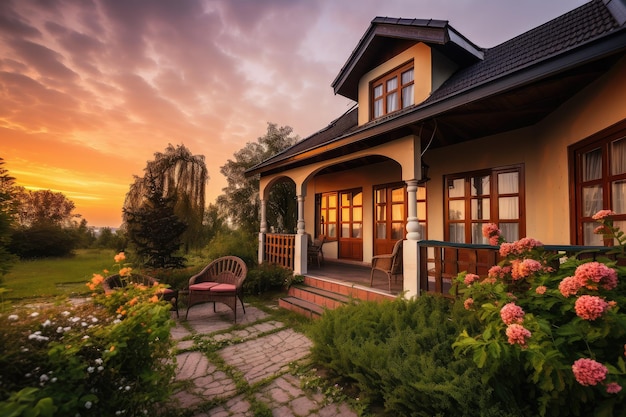The image captures a charming outdoor scene featuring a small, light orange-yellow house situated in the right corner, extending towards the right center at an angle. The house is accented by a dark tile roof, and it features multiple French door windows with wooden frames. A distinct characteristic of the home is its wraparound porch, accessible by three steps, and adorned with several chairs and a small table. An additional architectural detail includes a large window on the roof, hinting at a second story.

In front of the house lies a concrete pad with more chairs, and a cobblestone path leading away from it with grass growing between the stones. Surrounding the home is a well-maintained garden featuring an array of flowers in white, yellow, and pink, along with some bushes. The setting is further enriched by a green grassy lawn and a backdrop of trees.

The sky, depicting either a sunrise or sunset, contributes to the tranquil ambiance with its golden-orange hues and sparse clouds. In the distant background, there's a faint indication of a body of water, completing this picturesque scene.